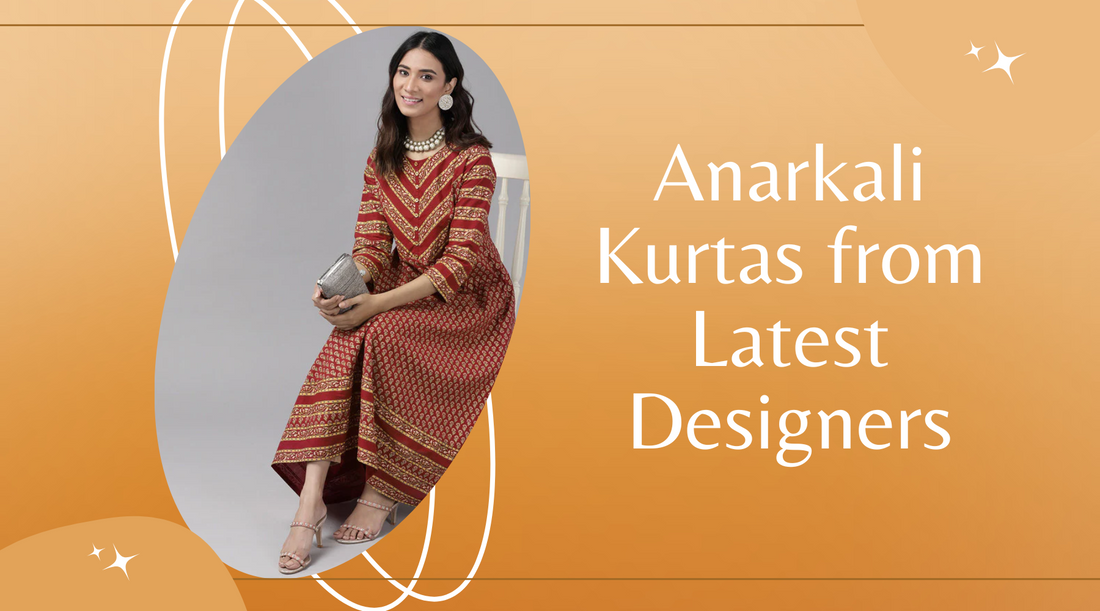The image is a print ad featuring a traditional South Asian woman wearing an Anarkali kurta, seated gracefully on a white wooden chair. The kurta, a long red garment with intricate golden designs, features striped patterns near the neckline, cuffs, and hem. The woman holds a grey clutch in her right hand and adorns herself with elegant silver jewelry, including a pearl necklace and large round earrings. She wears light-colored heeled sandals that appear to be embellished with jewels. The backdrop for this image is a light orange color, decorated with white stars and swirling lines, with a grey elliptical shape framing the seated woman. To the right, white text prominently reads: "Anarkali Kurta from Latest Designers." The woman, with her dark brown hair cascading down, smiles warmly, embodying Selina's stylish fashion essence.